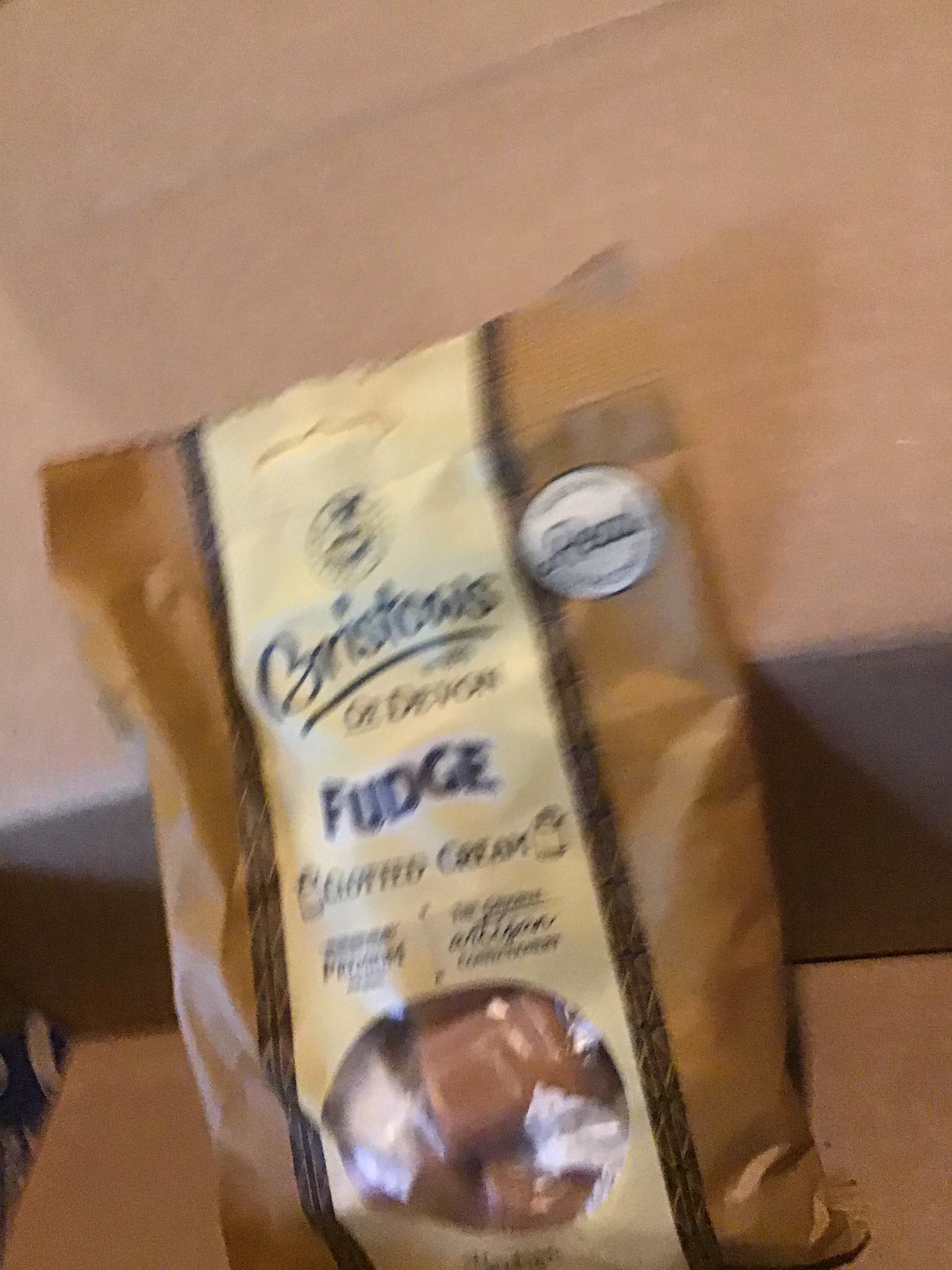The photograph showcases a blurry image of a Bristow's candy bag, prominently displaying the words "Bristow's of Devon" in cursive at the top. The package is primarily a brown paper bag adorned with a cream-colored label, featuring "fudge" in large black type and "clotted cream" beneath it. The bag includes a transparent circular section through which brown, individually wrapped square pieces of candy, resembling caramel squares, can be seen. The setup is on a light wooden tabletop against a wall that appears to have a faded pinkish beige hue, divided horizontally by a dark gray line. In addition, there are two vertical brown stripes and a vertical tan cream stripe on the plastic bag, which leans against the wall, further adding to the visual complexity of the background.